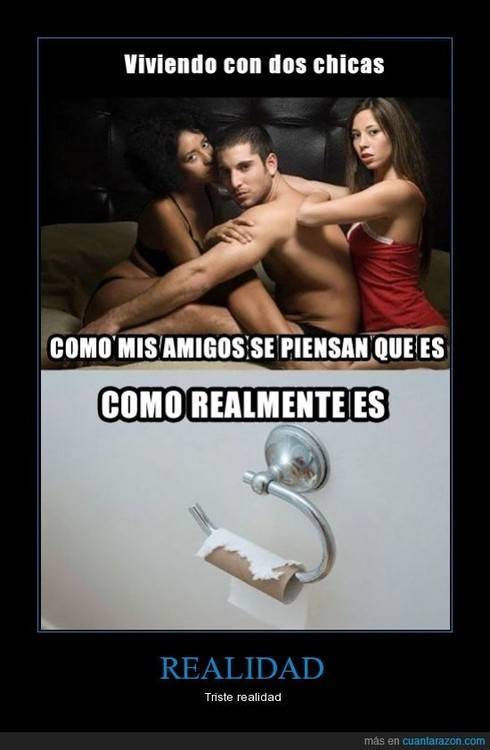The meme features a black background with two vertically aligned photographs and accompanying text in Spanish, exploring a humorous contrast. The top photograph shows a young man sitting on a bed in his underwear, flanked by two women. One woman massages his back while the other massages his bicep and kisses his head, suggesting a luxurious, pampered scenario. Above this image, the text reads, "Viviendo con dos chicas," and below it, "Como mis amigos se piensan que es romantes." The bottom photograph is of a nearly empty toilet paper roll hanging on a metal holder, depicting a starkly mundane reality. The text above this image states, "Como realmente es." Below both images, in blue and white text, it says, "Realidad Triste Realidad," emphasizing the contrast with a touch of irony. The bottom right corner bears the watermark “masquanta.com,” and the entire meme is framed by a subtle gray rectangular border at the top.